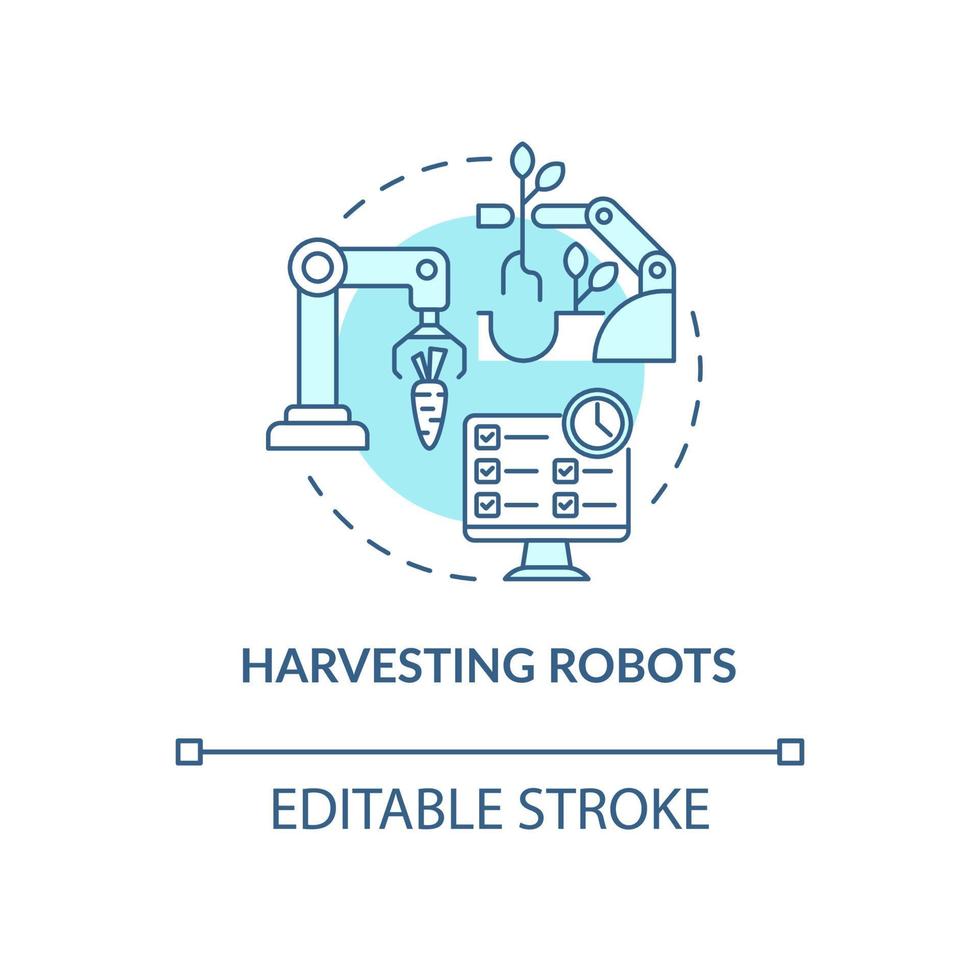The image features a detailed digital drawing against a white background, primarily rendered in shades of blue and light blue. Central to the composition is a large circle outlined with short blue dashes. Within this circle, interconnected by the dashed outline, are various mechanical and robotic devices depicted with intricate precision.

On the left, there is a machine with a white base stand, a light blue vertical bar topped by a circle, and an arm extending outwards resembling a faucet. Attached to the arm is a two-pronged device designed for gripping objects, interacting with a white carrot-like shape beneath it.

To the right, another device with a base and upright components includes an arm lifting a plant-like image. Adjacent to this is a stick figure with two legs and two heads, near a small tubular piece. Below the figure, a blue U-shaped line extends rightward, sprouting a stem with two light blue ovals above it.

At the bottom of the circle lies a screen-like element with a light blue base displaying a white board marked by columns of check marks and lines, along with a clock in the upper right corner. Central to the circle is a smaller blue circle, maintaining balance in the design.

Beneath this circular ensemble, large blue text reads "Harvesting Robots." Below this title is a horizontal line extended by squares at both ends, followed by the phrase "editable stroke" in significant blue writing. The entire design, composed of robotic elements, text, and stylized icons, maintains a cohesive blue and white color scheme, adding to the modern digital aesthetic of the image.